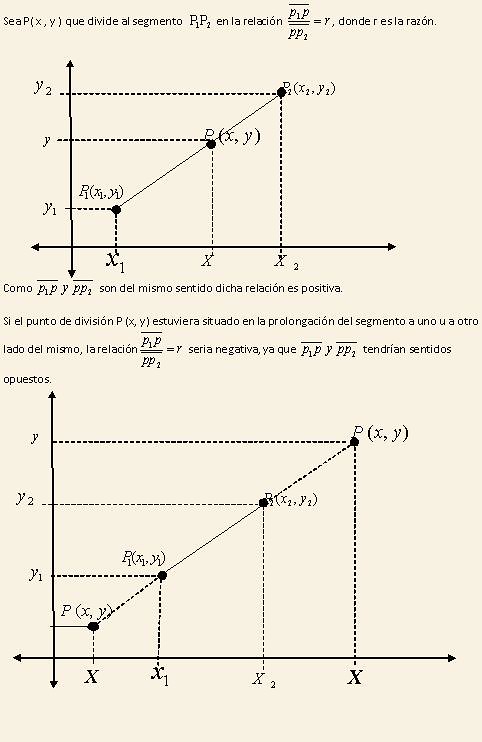This color photograph depicts a black and white diagram set against a creamy background, showing two mathematical graphs, one above the other. Each graph features clearly labeled X and Y axes with arrowheads indicating both directions. The diagrams contain diagonal lines extending from the lower left to the upper right. Notably, the X and Y axes are labeled with coordinates such as X1, X2, and X0. The text, written entirely in Spanish, includes several mathematical formulas and terms related to radii and segments, which are intermittently translatable to English. The top graph is slightly smaller, while the bottom graph is larger; both have black text and lines that stand out against the light-colored backdrop, forming a detailed illustration of mathematical relationships.